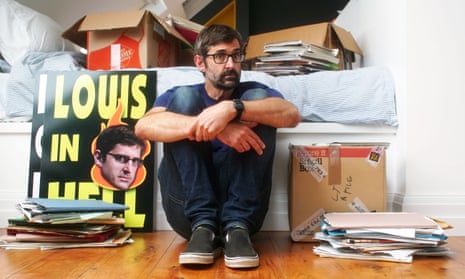In this detailed photograph, we see a man sitting on a light-colored wooden floor in what appears to be a cluttered room. He has short, brownish hair with a hint of gray, a black beard, and glasses. Dressed casually in a blue t-shirt, blue denim jeans, and gray sneakers, he sits with his legs pulled to his chest, arms wrapped around them, and appears to be looking off to his left. An Apple Watch adorns his left wrist.

To his left, there are posters leaning against the built-in bed, prominently featuring one that reads "Lewis in Hell" with an image of his face and flames in the background. Below these posters is a disorganized stack of papers and books. To his right, another stack of papers and books sits in front of a taped and labeled brown box, suggesting an ongoing packing effort. The bed behind him is messy, covered with boxes, magazines, and a blue bed covering with fluffy white pillows on the left side.

The setting seems to be a private space where the man might be preparing to move or simply overwhelmed by clutter. The overall scene captures a moment of introspection amid a backdrop of organized chaos.